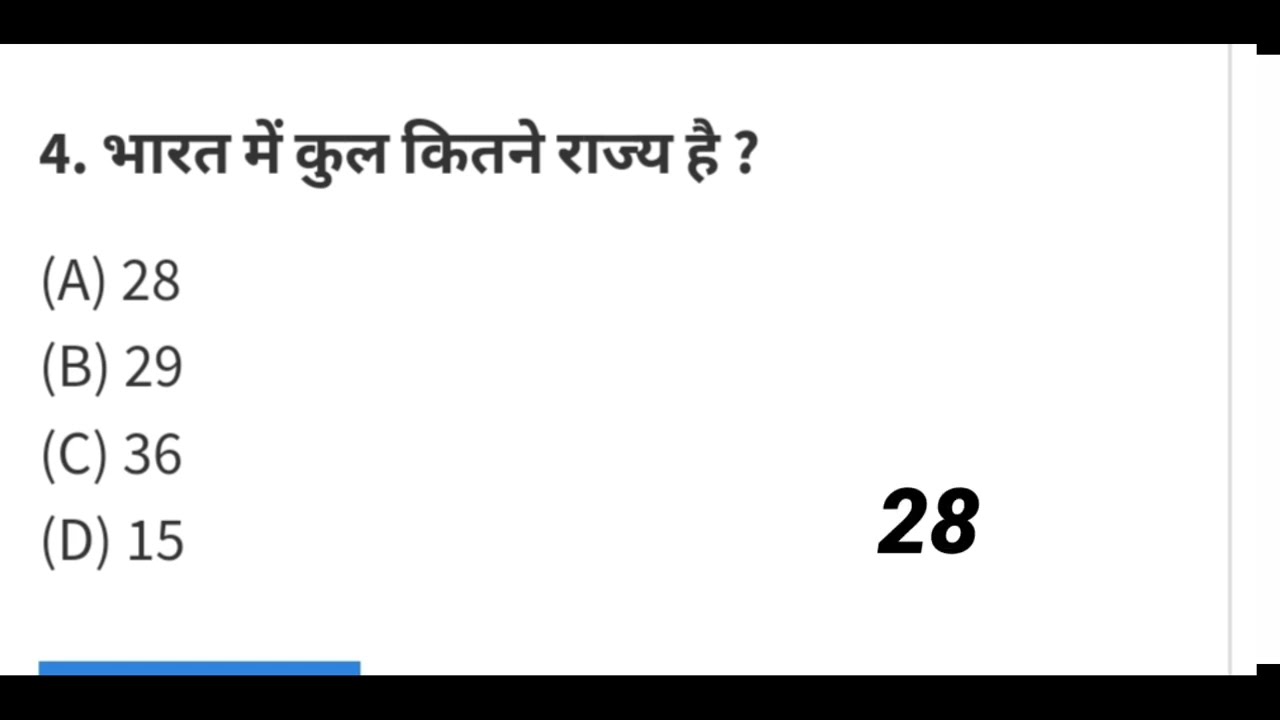This is an educational slide displayed on either a computer or a TV monitor. The primary background is white, featuring black text throughout. At the upper left-hand corner, there is the number "4" followed by a line of text in an unfamiliar script, likely Arabic, ending with a question mark. This is indicative of a question being posed. Below this, there are four bullet points labeled A, B, C, and D, each paired with a number: A. 28, B. 29, C. 36, and D. 15. The right-hand side prominently displays the number "28," which matches the option A, suggesting it might be the correct answer to the question. The lower left-hand corner of the slide features a blue stripe. Black bars run along the top and bottom of the image, framing the content and suggesting a structured format typical of educational materials.